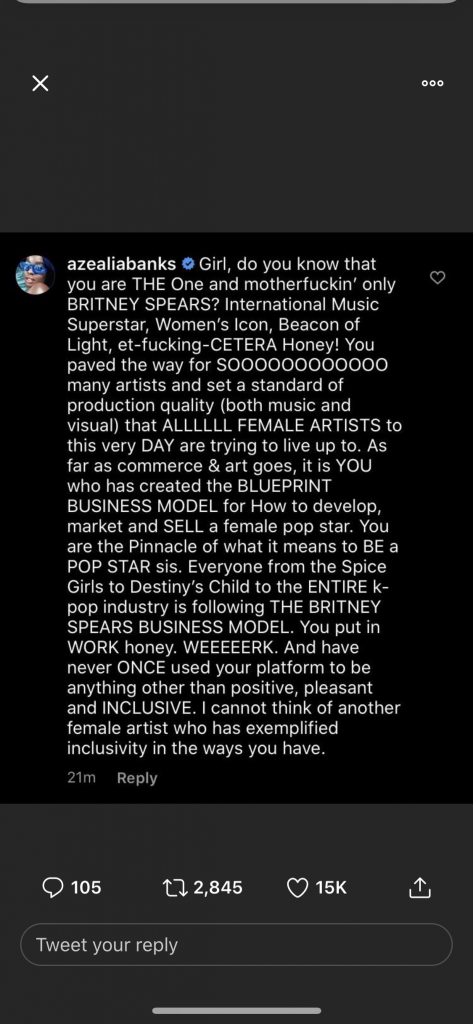The screenshot captures a social media post from a verified account of Azalea Banks, identified by a profile picture of a person wearing blue sunglasses. The post praises Britney Spears as a trailblazing icon in the music industry. The detailed message reads:

"Do you know that you are the one and motherfucking only Britney Spears, international music superstar, women's icon, beacon of light, Ed fucking cetra honey. You paved the way for so many artists and set a standard of production quality, both music and visual, that all female artists to this very day are trying to live up to. As far as commerce and art goes, it is you who has created the blueprint business model for how to develop, market, and sell a female pop star. You are the pinnacle of what it means to be a pop star sis. Everyone from the Spice Girls to Destiny's Child, the entire K-pop industry is following the Britney Spears business model. You put in work, honey, work, and have never once used your platform to be anything other than positive, pleasant, and inclusive. I cannot think of another female artist who has exemplified inclusivity in the ways you have."

The post was made 21 minutes ago and has garnered 105 responses, 2,845 shares, and 15,000 likes. There are interactive buttons for replying and tweeting a response. The screenshot interface includes a white 'X' and three white dots at the top, indicating additional options.